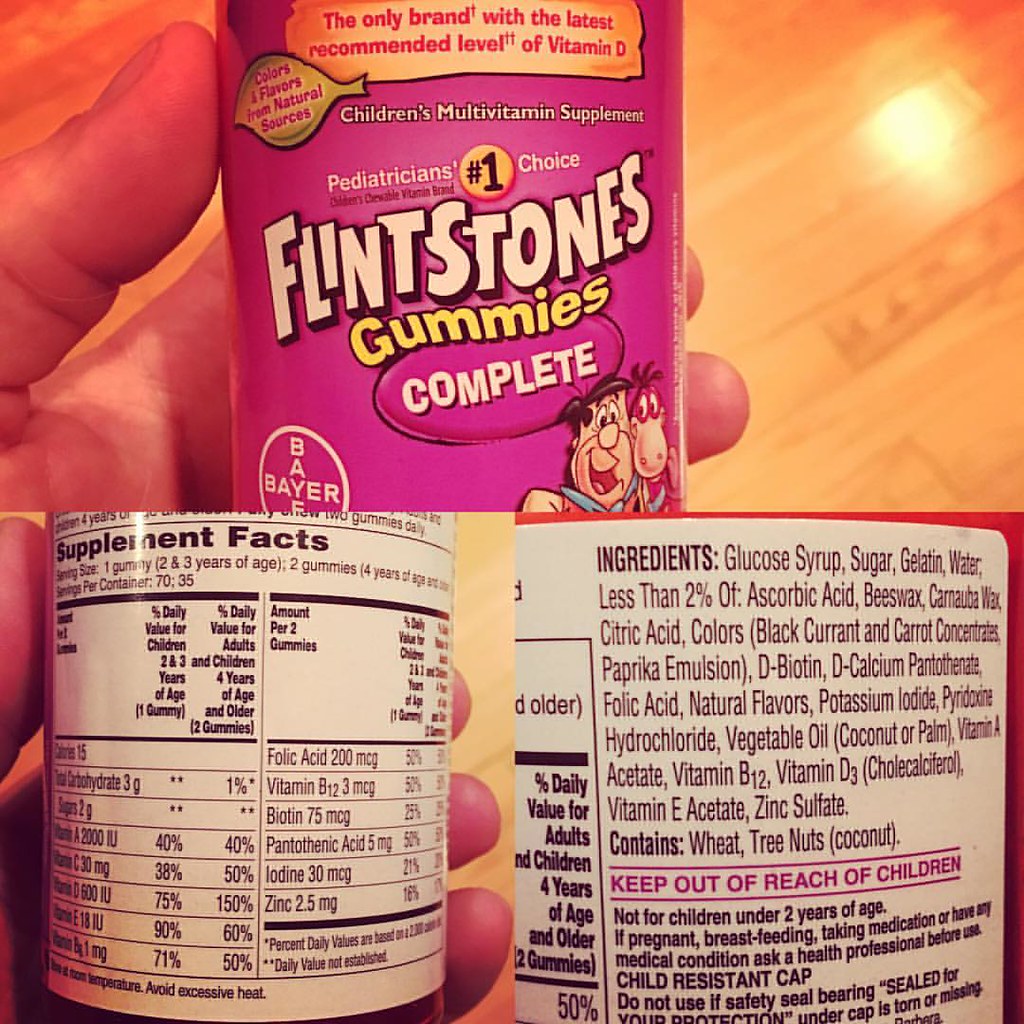This collage features three images combined into one, creating a detailed view of Flintstones Complete Gummies. 

The top section showcases a vertical rectangle photo of a white-skinned hand holding a purple jar of Flintstones Complete Gummies. The label prominently features colorful characters Fred Flintstone and Dino, adding a playful touch. The jar is held against a brown wood-grain floor, which has a light reflection in the bottom right corner.

The bottom section is split into two halves. On the left, there's a clear shot of the supplement facts, showing a hand holding the jar turned to display the black print on a white label. The right half zooms in on the ingredient list, where the text "Keep out of reach of children" stands out in purple. This close-up offers a detailed look at the label, emphasizing the product's safety instructions.